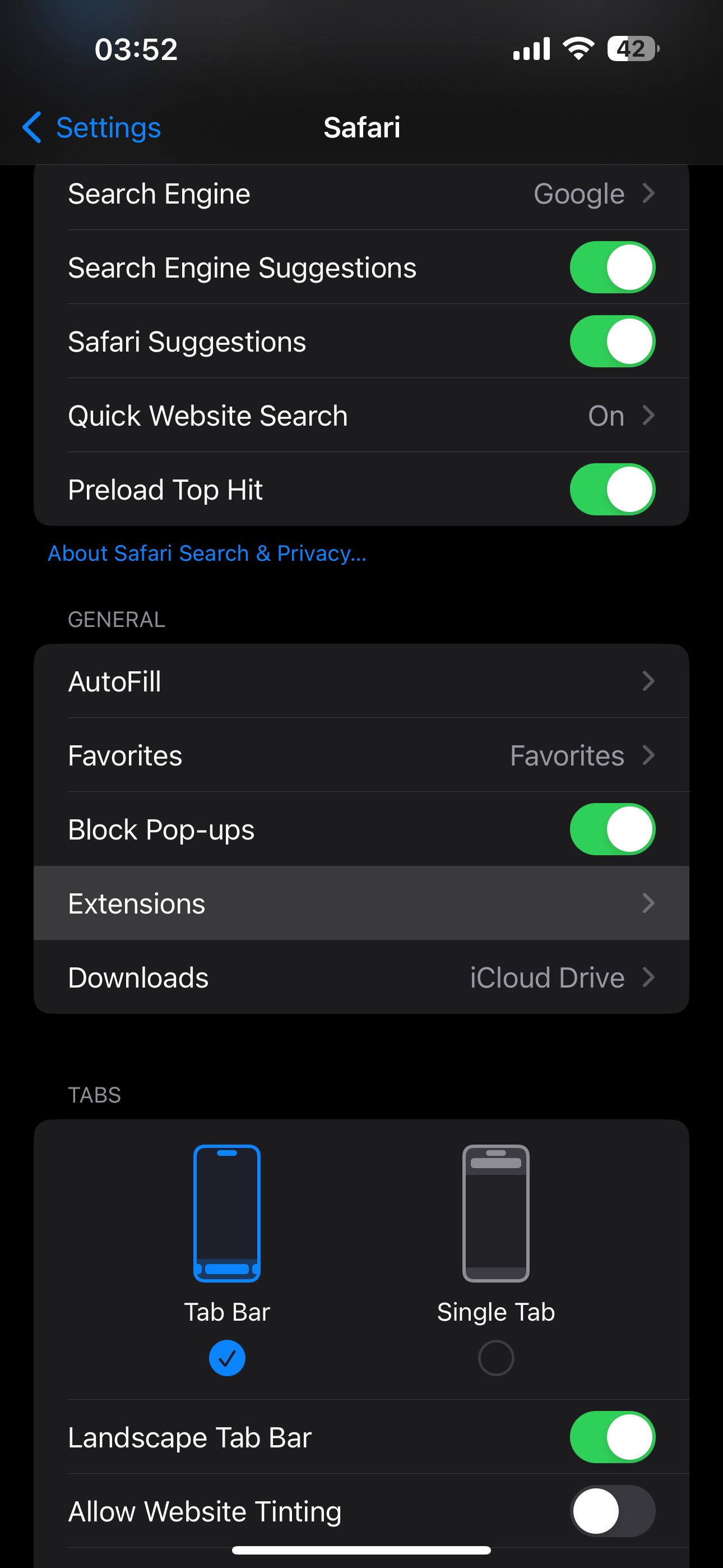This image is a vertical screenshot taken from a smartphone. The background is completely black and lacks any texture or dimension, presenting a solid flat appearance. 

In the top left corner, the time is displayed as 3:52, while the top right corner shows several icons—signal strength, Wi-Fi, and a battery icon indicating 42% battery life.

On the left side of the screen, the 'Settings' option is highlighted in blue, and the 'Safari' option appears in white at the center. Below, in white text, various Safari settings are listed:

- Google Search Engine Suggestions: toggled on (green)
- Safari Suggestions: toggled on (green)
- Quick Website Search: on
- Preload Top Hit: toggled on (green)

A blue link for "About Safari Search and Privacy" follows.

Under the 'General' section, we have:
- Autofill
- Favorites: displayed with a button
- Block Popups: toggled on (green)
- Extensions: highlighted in gray
- Downloads: shows "iCloud Drive"

Under the 'Tabs' section:
- Tab Bar: selected with a blue checkmark
- Single Tab: not checked
- Landscape Tab Bar: toggled on (green)
- Allow Website Tinting: not toggled on

This detailed layout captures the configuration and settings within the Safari browser on the smartphone.